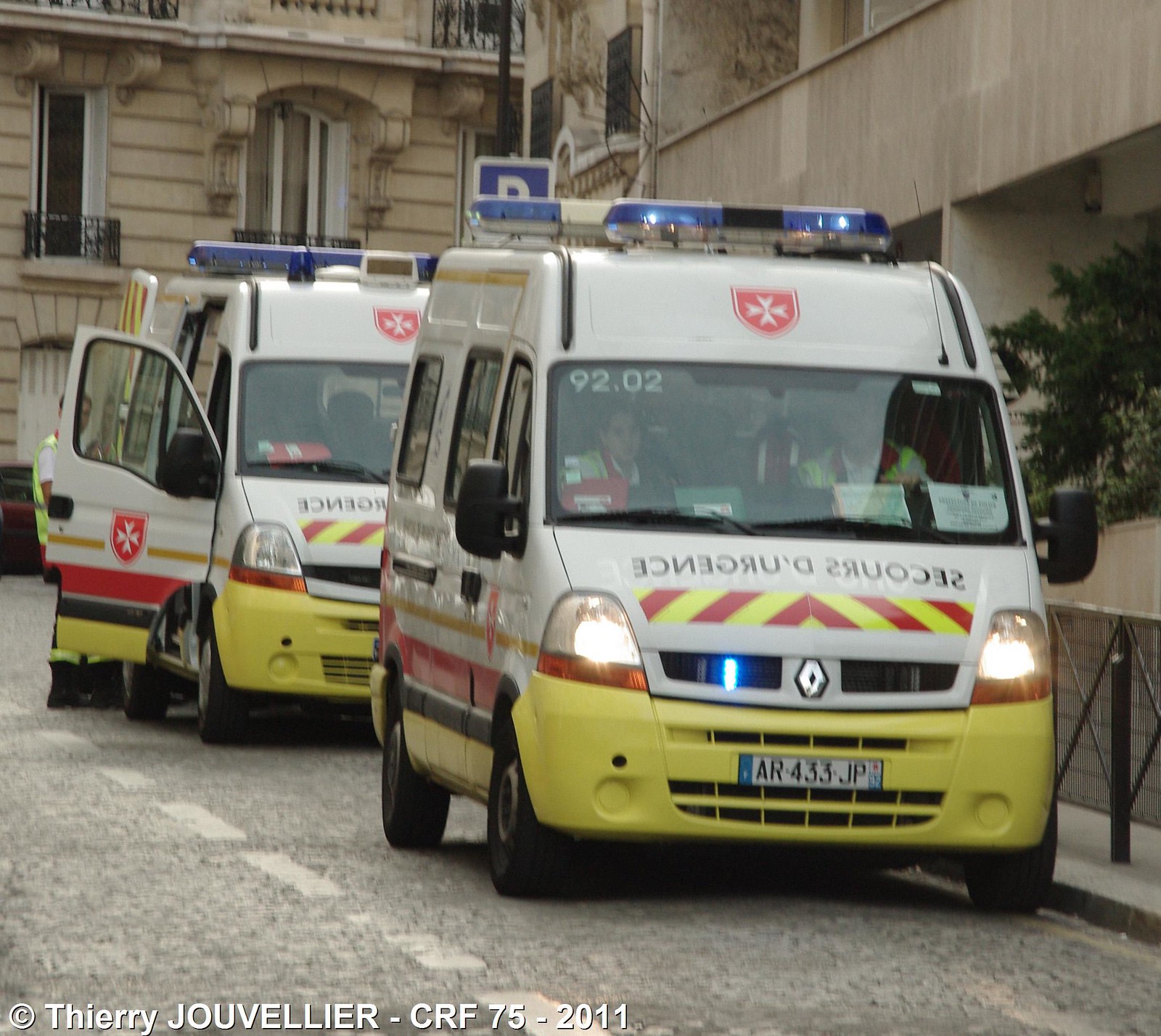In this 2011 photograph by Thierry Juvelier, two French ambulances are depicted on a city street, with the scene suggesting a sense of imminent activity. The ambulances, primarily white with yellow bumpers, are emblazoned with the text "Secours d'Urgence" and the red cross on their roofs. The ambulance in the front has its sirens and blue lights activated, while the rear vehicle has its door open, indicating recent or ongoing preparations for departure. Both vehicles have a French license plate, such as "AR 433 JP". The photograph captures the ambulances amidst old residential buildings, characterized by their concrete or stone construction, situating the scene in an everyday urban setting in France.